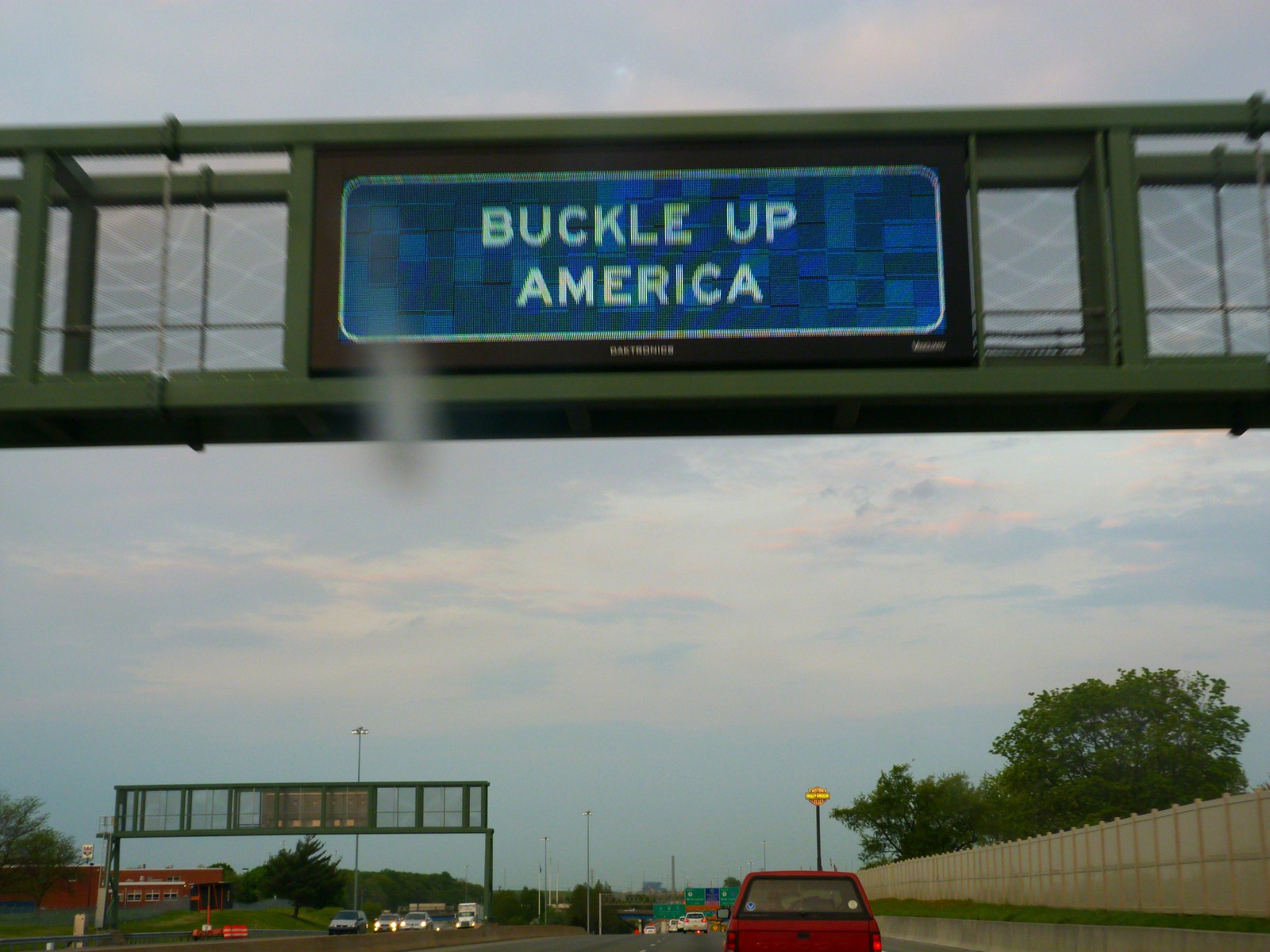The image is a first-person point-of-view photograph taken from within a moving car on a freeway. The camera is slightly tilted upward, capturing the scene through a windshield that has a blur or piece of dirt near the top left corner. The overcast, cloudy sky sets a gray tone for the scene. Prominently, there is an overhead signage structure with big green metal bars supporting an LCD screen. The screen has a checkered dark blue and purple background, bordered in white with bold, capitalized white text reading "BUCKLE UP AMERICA." Directly ahead, on this three-lane highway, a red pickup truck is visible, with its lights on. The freeway is divided by a barrier, with another three lanes for oncoming traffic to the left. A large barrier wall runs along the right side of the road, and streetlights and bits of buildings can be seen in the distant horizon.